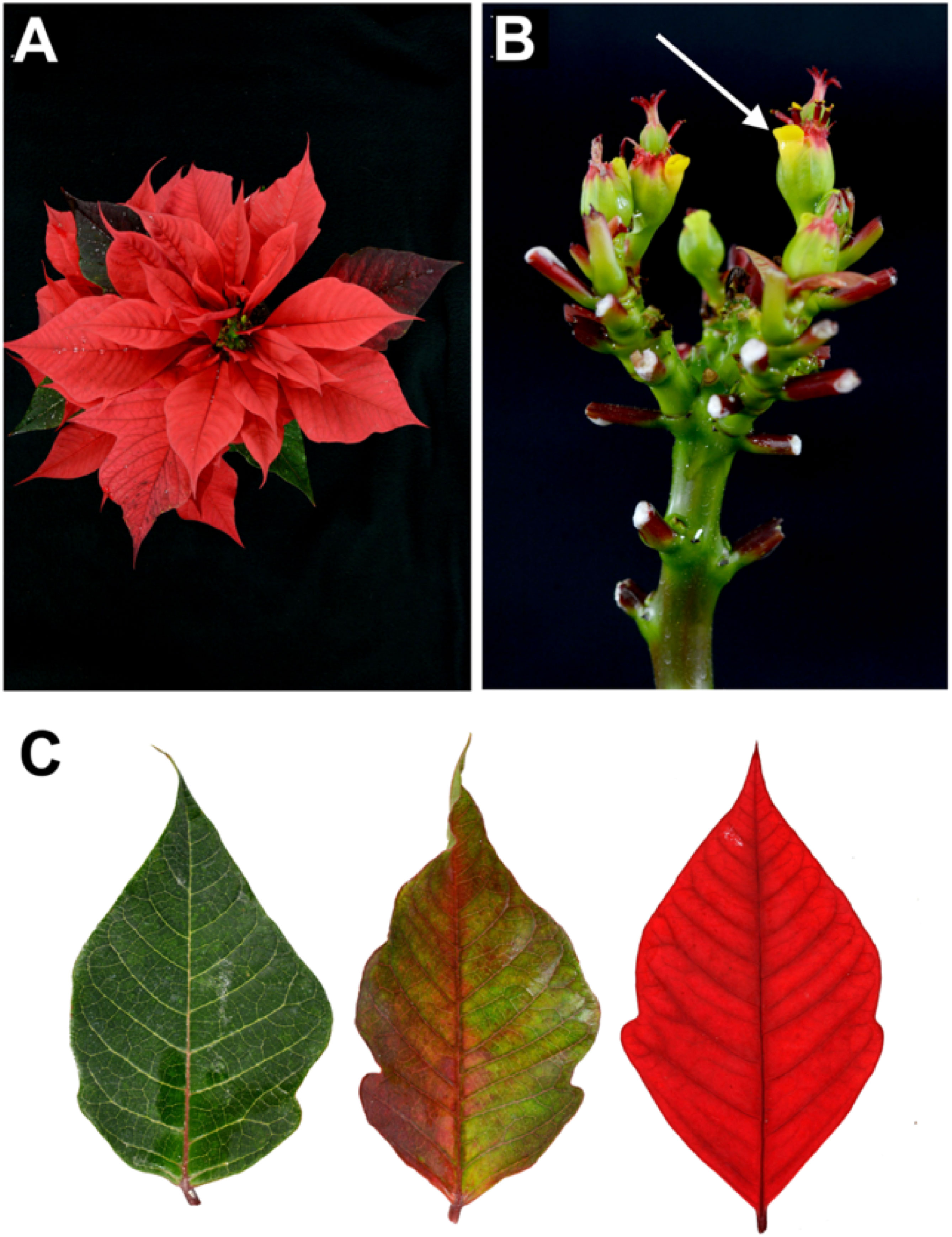The image provides a detailed illustration of poinsettias, broken into three labeled sections: A, B, and C. Section A, located in the upper left-hand corner, is a black rectangle showcasing an overhead view of a poinsettia flower in a light red hue. Section B, positioned immediately to the right of A, is also a dark rectangle of similar size, featuring a green stem with red-tipped buds at the ends of its branches. A white arrow points to one of these buds, indicating the point of new growth. Section C, spanning the entire bottom half of the image on a white background, depicts poinsettia leaves in three different stages of color transformation. The leaf on the left is dark green, the middle leaf is transitioning with light green and pink splotches, and the leaf on the right is fully pink. The illustration highlights the poinsettia's growth process and seasonal color change, emphasizing the plant's ability to regenerate and transform from year to year.